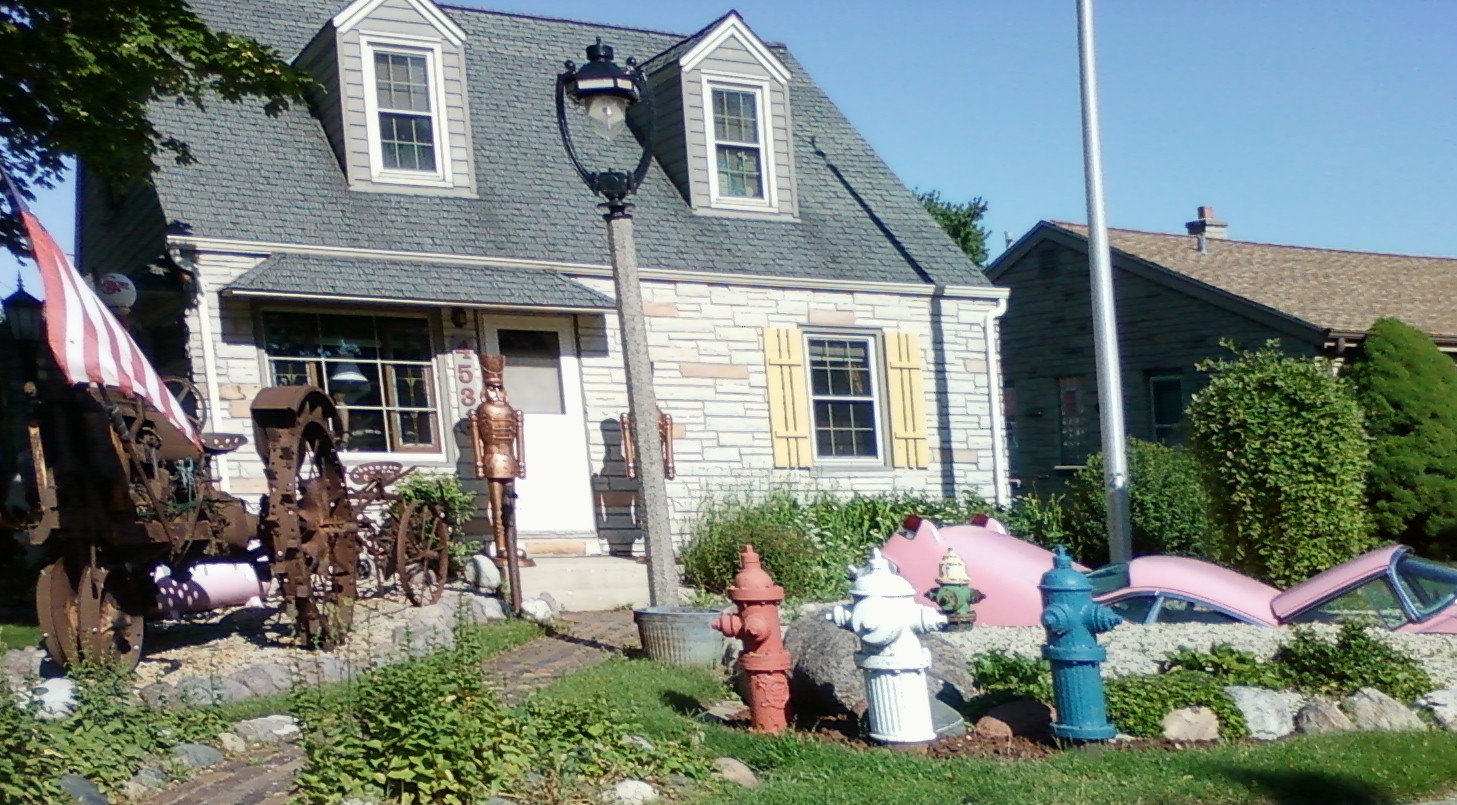This photograph showcases a unique residential homestead featuring a gray, colonial-style, two-story house adorned with a multicolored, slate wall exterior and a green roof. The front yard is visually striking, containing a lush patch of green grass interspersed with gravel and various decorative elements. Central to the yard are four fire hydrants, each distinctively colored: a slender red, a wider white, a thin blue, and a green with a yellow cap.

Prominently displayed is an artistic sculpture made from a pink car, seemingly broken and submerged into the ground, with both the back and front ends sticking out. An American flag stands tall, mounted on what appears to be an old rusty tractor or possibly a cart, evoking a historical feel with its cannon-like wheels.

Guarding the front door are two robust nutcracker statues, which add a festive or whimsical touch to the entrance. The yard is further complemented by a variety of bushes, rock formations, and baskets that contribute to the rustic charm of this eclectic homestead. The image also partially reveals a neighboring one-story brown house peeking from behind thick shrubbery.